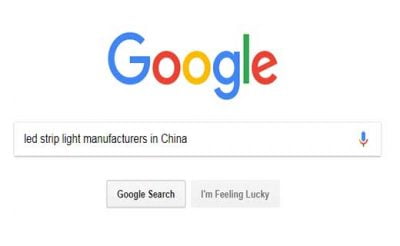The image depicts Google's search homepage set against a plain white background. Prominently centered at the top is the iconic "Google" logo, with each letter in a distinct color: the 'G' in blue, the first 'O' in red, the second 'O' in yellow, the second 'G' in blue, the 'L' in green, and the 'E' in red. Below the logo, there's a search bar containing the query "LED strip light manufacturers in China" in black text. Underneath the search bar are two light gray rectangular buttons with black text: "Google Search" on the left, which is highlighted, and "I'm Feeling Lucky" on the right. The image encapsulates a typical Google search page in action, focusing on the user’s query about LED strip light manufacturers in China.